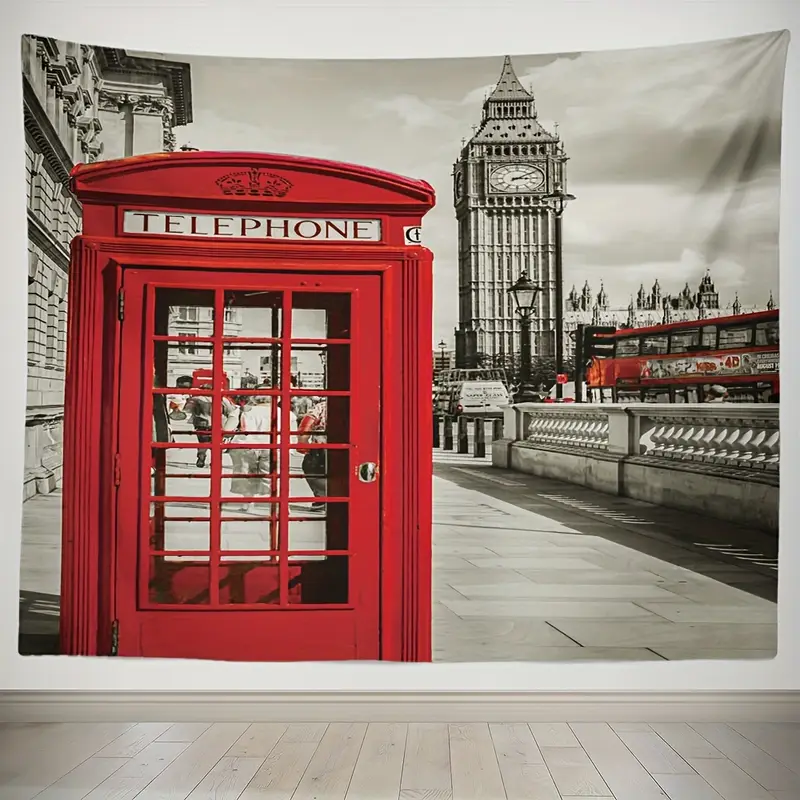The image depicts a wall tapestry featuring a black and white photograph of an outdoor scene in London, prominently hung on a white wall with light-colored wood flooring below. Dominating the view is a bright red British telephone booth on the left, contrasting starkly against its monochrome surroundings. Behind the booth, people can be seen walking leisurely. Towards the center-right of the tapestry is a somewhat squished depiction of Big Ben, suggesting the entire scene might have been compressed, making elements appear flattened. A red double-decker bus stands out on the right side, and further back, faintly visible are the architectural elements of Parliament. A peculiar addition to the scene is a red boat on the Thames, breaking the grayscale aesthetic. The sky above is light with some clouds, and the far background shows what appears to be a mixture of street slums and castle-like structures, adding to the bustling ambiance of the streets below.